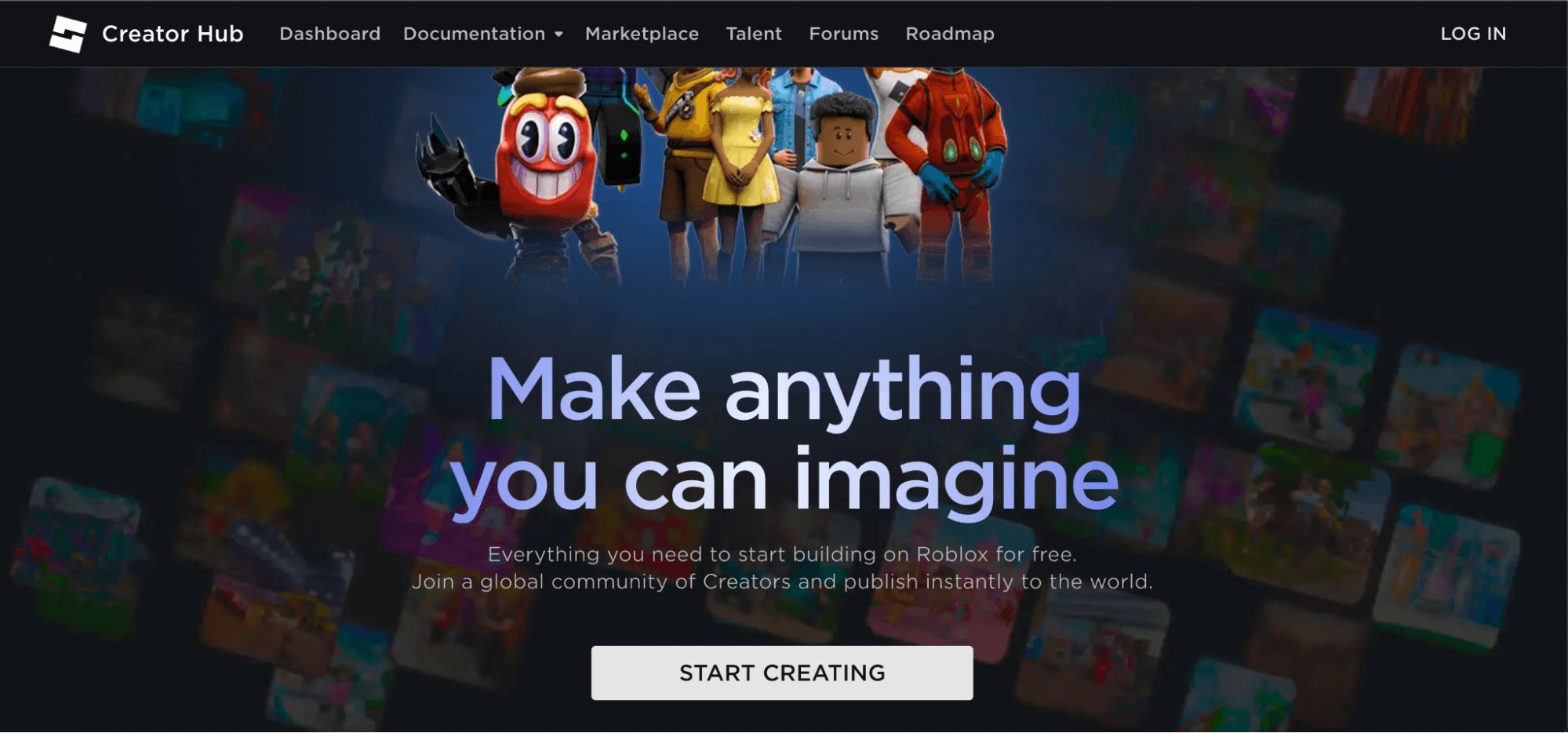The image is a horizontally oriented graphic with a detailed composition. The top portion features a black background. On the upper left corner, there's a small icon followed by the text "Creator Hub" in bold white letters. Adjacent to this, moving right, are the menu options: "Dashboard," "Documentation" with a downward arrow suggesting a dropdown menu, "Marketplace," "Talent," "Forums," and "Roadmap." On the far right is a "Login" button.

Beneath this interface, the background transitions into a collage of digitally-created images, some partially obscured, giving a sense of a creative, dynamic environment. This collage has a faded overlay effect to ensure focus remains on the essential text and icons in the foreground.

In the center of this creative backdrop, in blue bubble letters with a blue-white ombre effect, the inspirational phrase "Make Anything You Can Imagine" stands out prominently. Directly below this tagline, a white text description offers further encouragement: "Everything You Need to Start Building on Roblox for Free. Join a global community of creators and publish instantly to the world."

At the bottom of the image, a call-to-action is presented in a white rectangular box. Inside, in bold black uppercase letters, the text "START CREATING" invites viewers to embark on their creative journey.